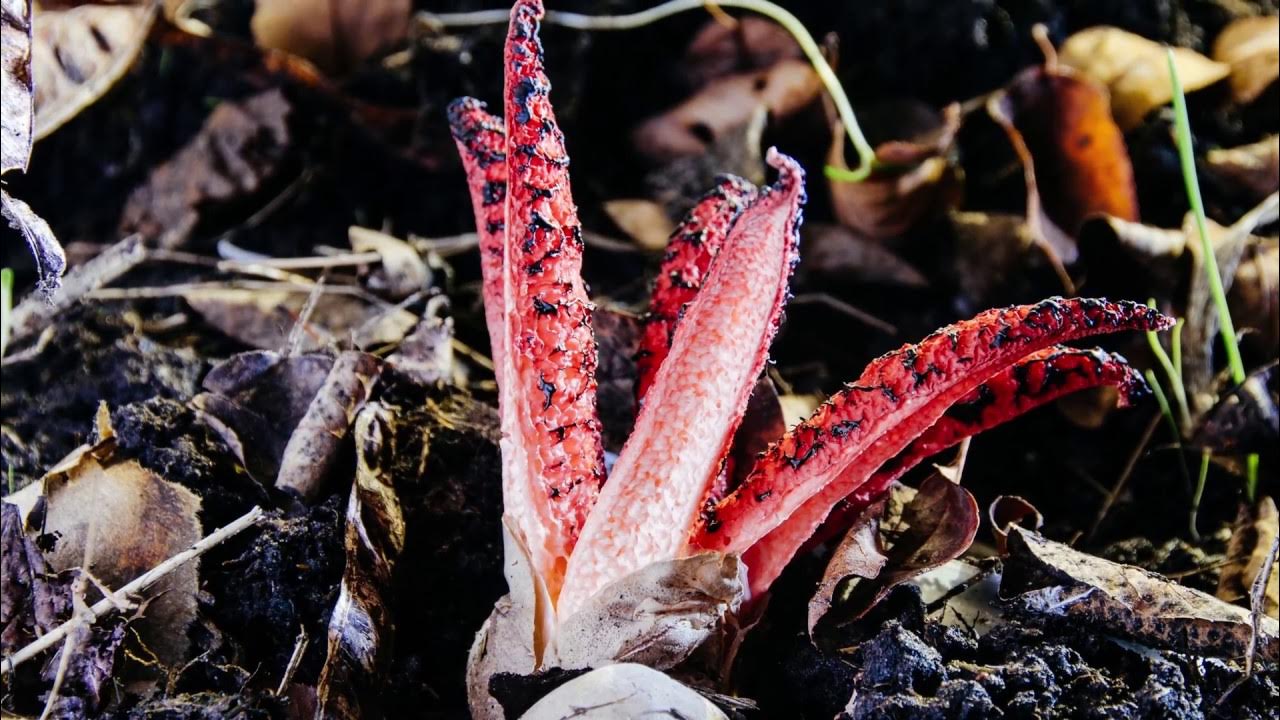The image is a close-up shot of soil, showcasing a peculiar central object that is identified as a unique type of mushroom. The main object has an unusual, almost phallic shape, with several mushroom stalks emerging from one spot. The mushrooms are predominantly white at the base, transitioning to shades of red with black splotches towards the tips, which include six tentacle-like extensions that give it an octopus-like appearance. The central mushrooms are surrounded by a background of dead leaves, vines, and some green grass sprouts, along with other plant debris on the dark brown to black soil. The vivid colors in the image include black, brown, dark brown, varying shades of green and brown, peach, red, white, and a hint of purple. The overall impression is one of a strange and somewhat vibrant growth amidst decaying plant matter. There is no text visible in the photograph.